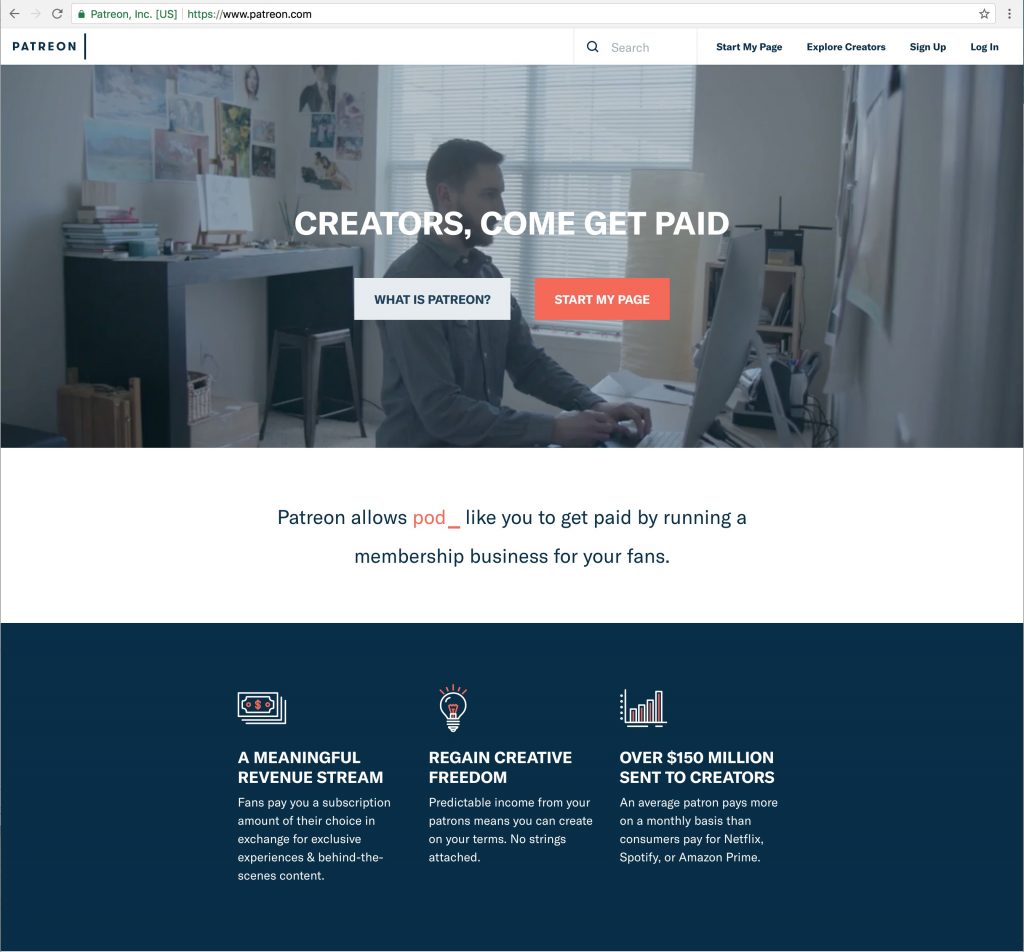This is a detailed description of a webpage from Patreon, featuring multiple visual and textual elements that emphasize the platform's offerings for creators. 

The webpage is vertically oriented and rectangular. In the upper left corner, the Patreon logo is visible, though the font color is difficult to discern. The website's URL is also displayed in the search bar at the top of the page, initially in green, followed by black.

The top section of the page has a horizontal rectangular banner with the large, white, all-capitalized text: "CREATORS, COME GET PAID," positioned centrally. Below this are two smaller horizontal rectangles. The first, in white with a blue font, asks "What is Patreon?" The second, slightly smaller and orange, has white text saying "Start my page."

The background image is softly faded and depicts a man working at a computer desk, facing the right edge. Behind him, another desk with a chair and various papers pinned to the wall adds to the workspace ambiance.

Beneath this image, blue text states "Patreon allows," followed by "pod_" in orange font. The complete sentence, "Patreon allows pod_ like you to get paid by running a membership business for your fans," is partly stylized with an orange underscore.

The bottom section of the page mirrors the image section in size and features three consecutive messages, each accompanied by distinct icons:
1. "A MEANINGFUL REVENUE STREAM" (white, all caps). Below, it says, "Fans pay you a subscription amount of their choice in exchange for exclusive experiences and behind the scenes content," with a dollar bill icon above.
2. "REGAIN CREATIVE FREEDOM" (white, all caps). Below, it states, "Predictable income from your patrons means you can create on your terms, no strings attached." A light bulb icon accentuates this section.
3. "OVER 150 MILLION SENT TO CREATORS" (white, all caps). Below, the text reads, "An average patron pays more on a monthly basis than consumers pay for Netflix, Spotify, or Amazon Prime," paired with a bar graph icon.

Each icon is white with orange accents, harmonizing with the overall design scheme of the webpage.